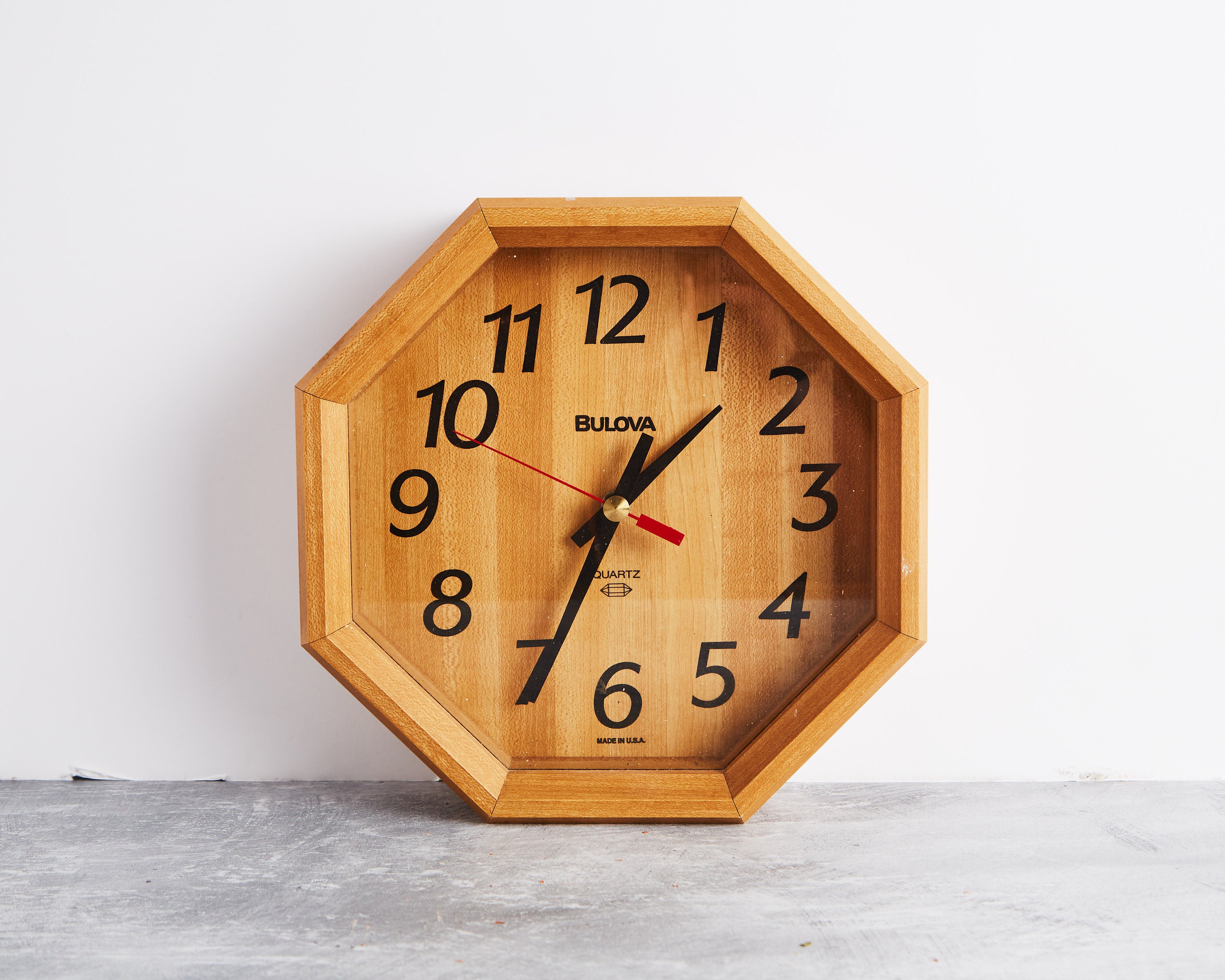This photograph captures an indoor scene featuring a wooden, hexagonal wall clock set against a white background and a gray, concrete-like surface. The clock, crafted from light-colored wood, prominently displays the brand "Bulova" in black lettering beneath the number 12, and the word "Quartz" accompanied by a stylized quartz crystal symbol above the number 6. Additionally, "Made in USA" is inscribed in black font below the number 6. The clock face includes black numeric hour markers from 1 to 12 and is equipped with black minute and hour hands, along with a red second hand. The hands are anchored at the center by a brass-colored mechanism, with the hour hand positioned between 1 and 2, the minute hand on 7, and the second hand on 10. This detailed timepiece leans against a white wall, resting on a gray surface.